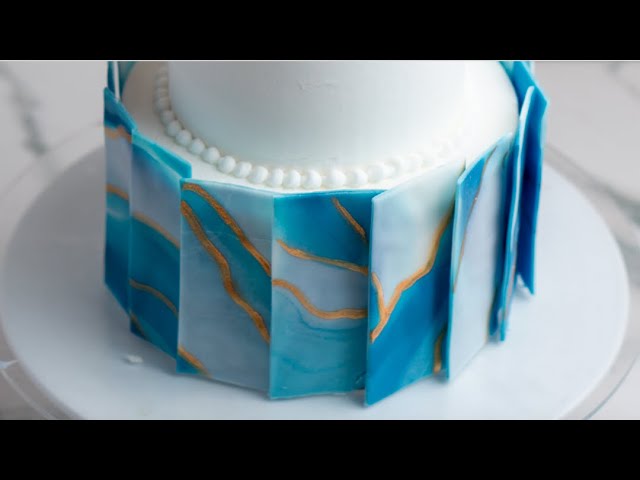This photograph, taken by a photographer without the aid of AI technology, captures an exquisite wedding cake as its central subject. This cake, a masterful creation, is presented on a pristine white dish, elegantly placed atop a table. The image features distinct black borders at both the top and bottom, framing the scene. The cake itself is adorned with intricate designs, showcasing a harmonious blend of colors including white, blue, gold, black, and ivory. The detailed embellishments and overall composition exemplify both artistry and craftsmanship, making the cake not just a dessert, but a visual masterpiece. The photographer has skillfully made the wedding cake the focal point of the image, ensuring it commands the viewer’s attention.